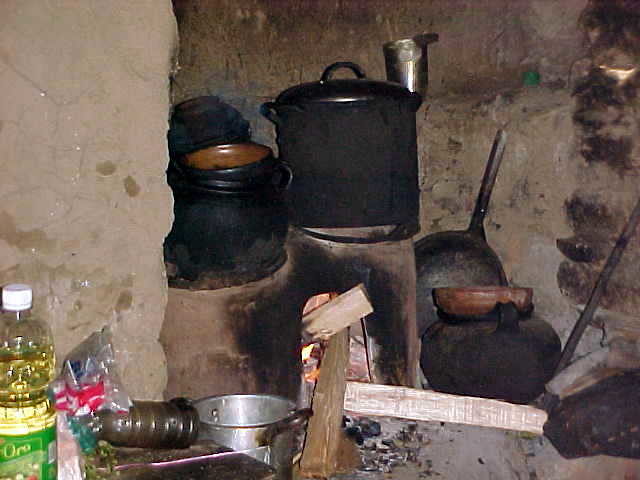This color photograph showcases the interior of an old home, focusing on a vintage fireplace used for cooking in the 1800s. The centerpiece is a dome-shaped fireplace with a flat top, sporting a blackened door and soot-streaked, uneven brick walls. Inside and around the fireplace, there's a collection of black pots and cast-iron skillets of various sizes, some placed inside the fireplace itself and others atop it. The beige stone wall in the background is marked by smoke stains and has an intricate structure that includes an indent on the left side. In front of the fireplace, firewood is neatly stacked, indicating preparations for building a fire. 

To the side of the fireplace, a steel table holds a tall bottle of cooking oil with a white cap and a green label, along with a plastic bag and a brown and black plastic water bottle. A stainless steel pot with dark handles sits nearby, accompanied by a round black pot cover with a copper bowl on top. A large black frying pan leans against the wall, and a silver pail rests on a ledge above. The scene is rich with historic charm, showing the well-used tools and utensils of a bygone era.